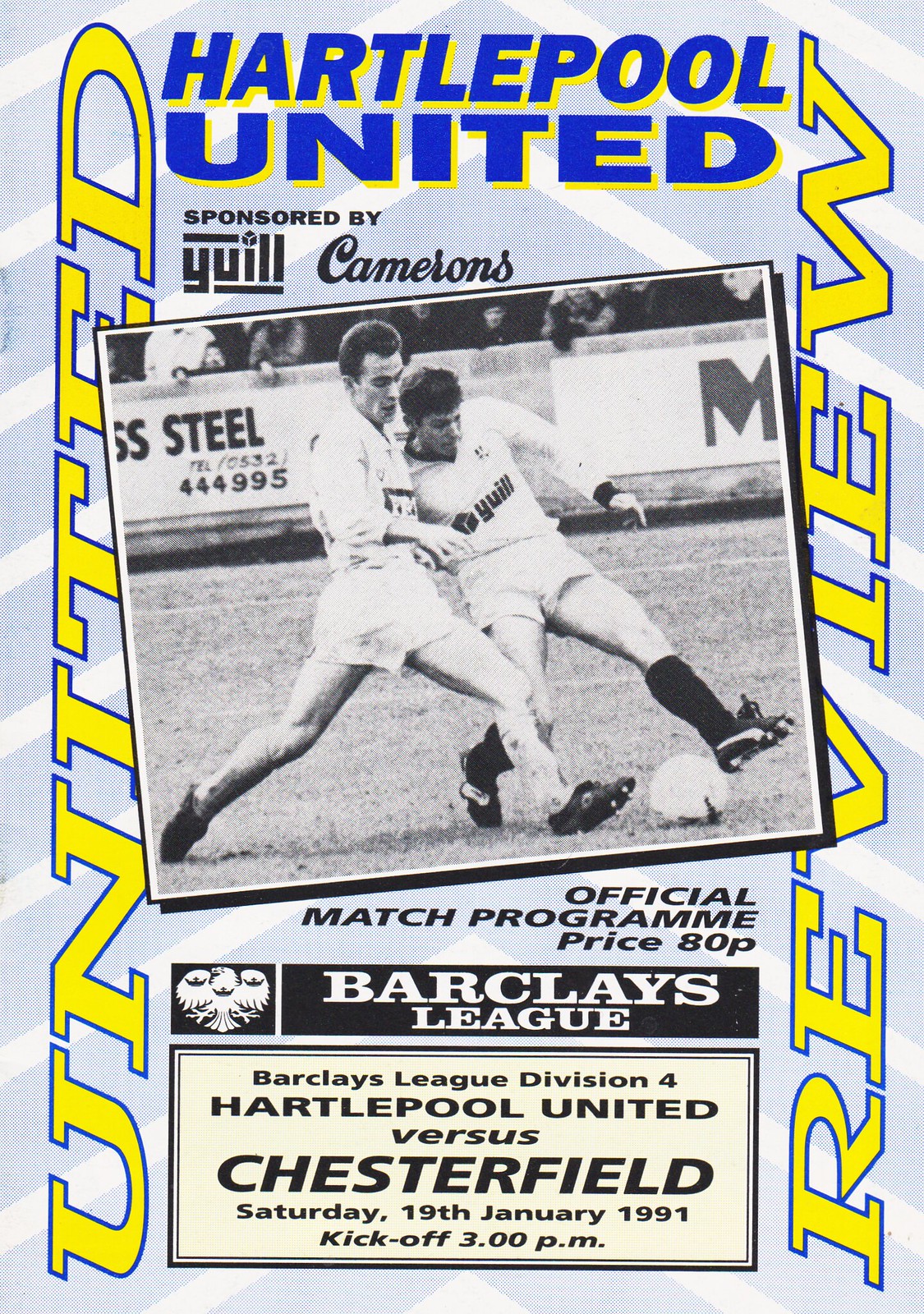The image is of the cover of an official match program for a football game between Hartlepool United and Chesterfield, scheduled for Saturday, January 19th, 1991, with a kickoff at 3 p.m. At the top of the program, "Hartlepool United" is prominently displayed in blue and yellow letters, sponsored by Camerons. The center of the cover features a dynamic, slightly tilted image of two players from opposing teams battling for the soccer ball, with some spectators visible in the background. Below this action shot, the text reads: "Official Match Program, Price 80 pence," followed by "Barclays League, Barclays League Division 4, Hartlepool United vs. Chesterfield." Flanking the central image, the words "United" and "Review" run vertically along the left and right sides, respectively, in yellow letters. This program encapsulates the anticipation and excitement for the forthcoming match.